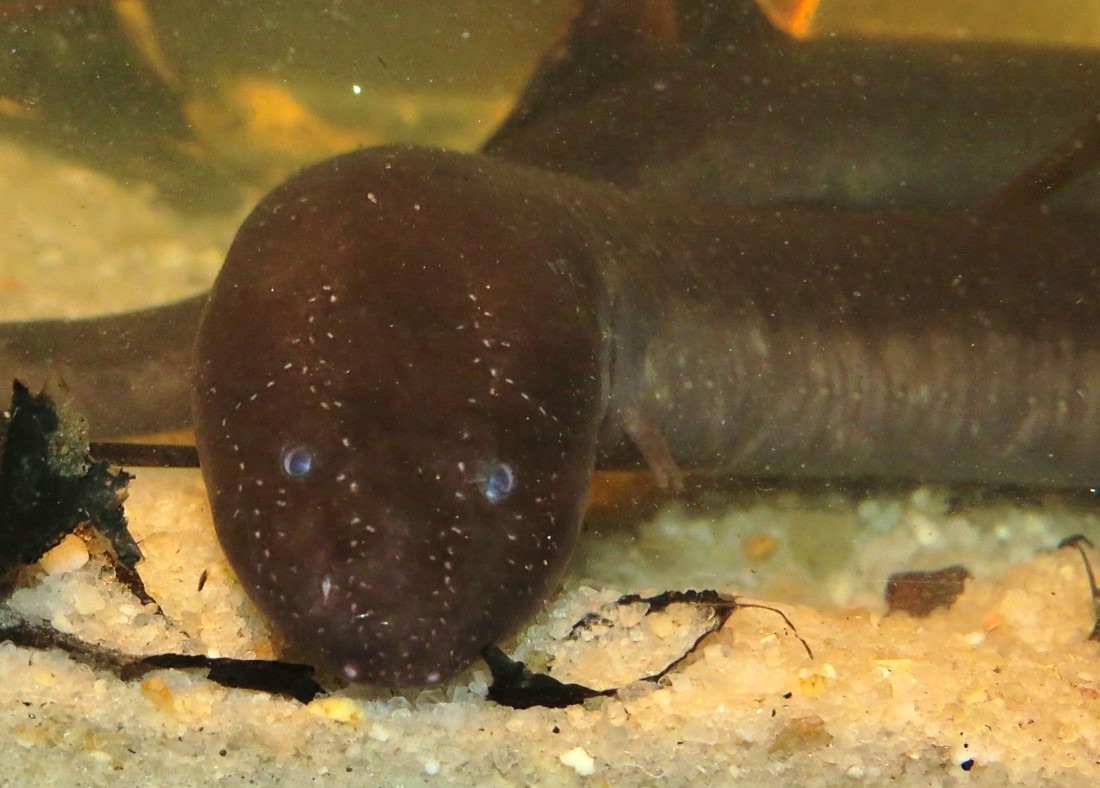This detailed underwater photograph captures a salamander-like creature, possibly an amphibious reptile, resting on a light-colored, sandy, grainy substrate. The creature, with its dark brown body and slightly gray belly, is central to the image, which is zoomed in on its face. It has two small, short arms and blue eyes that stand out against its murky environment. The creature also has black feelers or some kind of black material protruding from or near its mouth. The background of the photograph is slightly blurry, indicating either a murky aquatic setting or an aquarium. Above the substrate, which appears to be composed of light white and yellow crystals, there's a long, barrel-shaped fish visible in the background. This fish has silvery gray scales with a dorsal fin, and it seems to float above or rest on the substrate at the bottom of the scene. The overall setting is enveloped in a hazy aquatic atmosphere, with subtle hints of water plants or growth in the upper left corner.